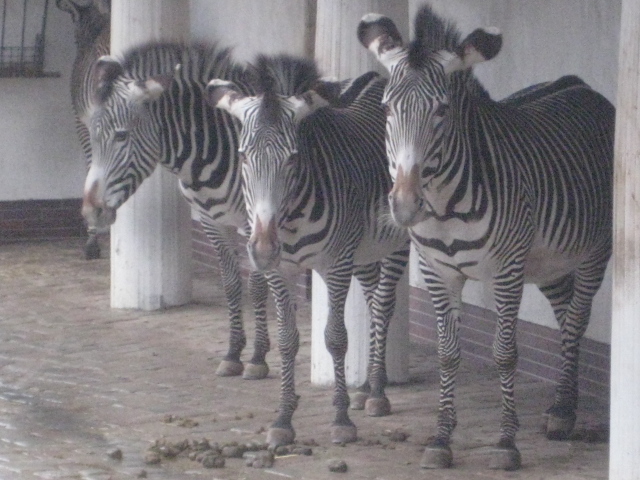The photograph, somewhat grainy and faded, features three zebras standing side by side on a roughly tiled or paved outdoor floor, which has patches of dirt or zebra dung. These zebras are predominantly black and white with light brown muzzles, and they sport tufted, upright manes. Each zebra has unique stripe patterns, which widen on their bodies and appear on their long, skinny legs. They are generally facing the camera, though only the central zebra looks directly into it. Behind them, a building with a white exterior and two large, fluted white columns is visible, flanked by a wall with a brick base approximately four or five bricks high. There's also a fourth zebra in the background, partially obscured, facing away from the camera. Additionally, a hanging basket can be seen on the left side of the wall. The overall palette of the image, although likely originally in color, appears washed out, lending it a black-and-white or grayscale look.